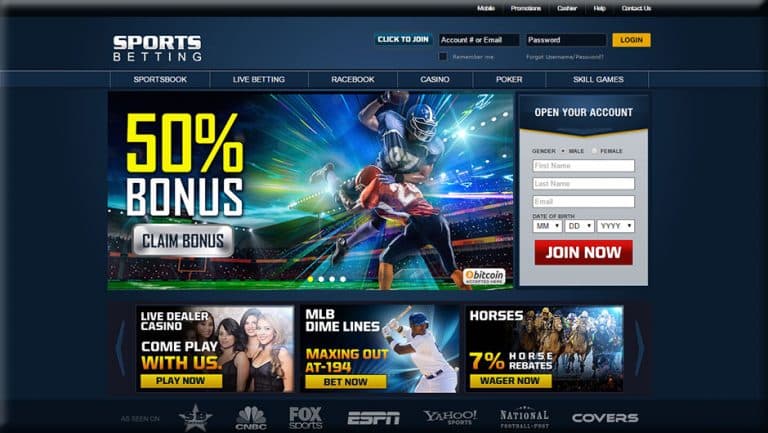The image showcases a screenshot of a sports betting website displayed on a computer screen. The website's interface features a dark blue background, complemented by a black navigation bar at the top displaying various menu options such as "Promotions," "Careers," "Help," and "Contact." Below the navigation bar, the website clearly states "Sports Betting" in white text, accompanied by a "Click to Join" call-to-action. 

Users are prompted to log in with their account and password through a login button characterized by black text on a vibrant yellow background. The site offers a variety of betting options listed in white text, including Sportsbook, Live Betting, Racebook, Casino, Poker, and Skill Games. A prominent section showcases a cartoonish image depicting players in a brightly lit stadium, highlighting a promotional offer. The text within this promotional area reads "50% Bonus," with "50%" in bold yellow text, while "Bonus" and "Claim Bonus" are in white text. 

To the side of the promotional graphic, there's an "Open Your Account" section where new users can enter their email address, date of birth, and other required details. This section concludes with a "Join Now" button, styled with white text on a red background, urging visitors to register and start using the site.